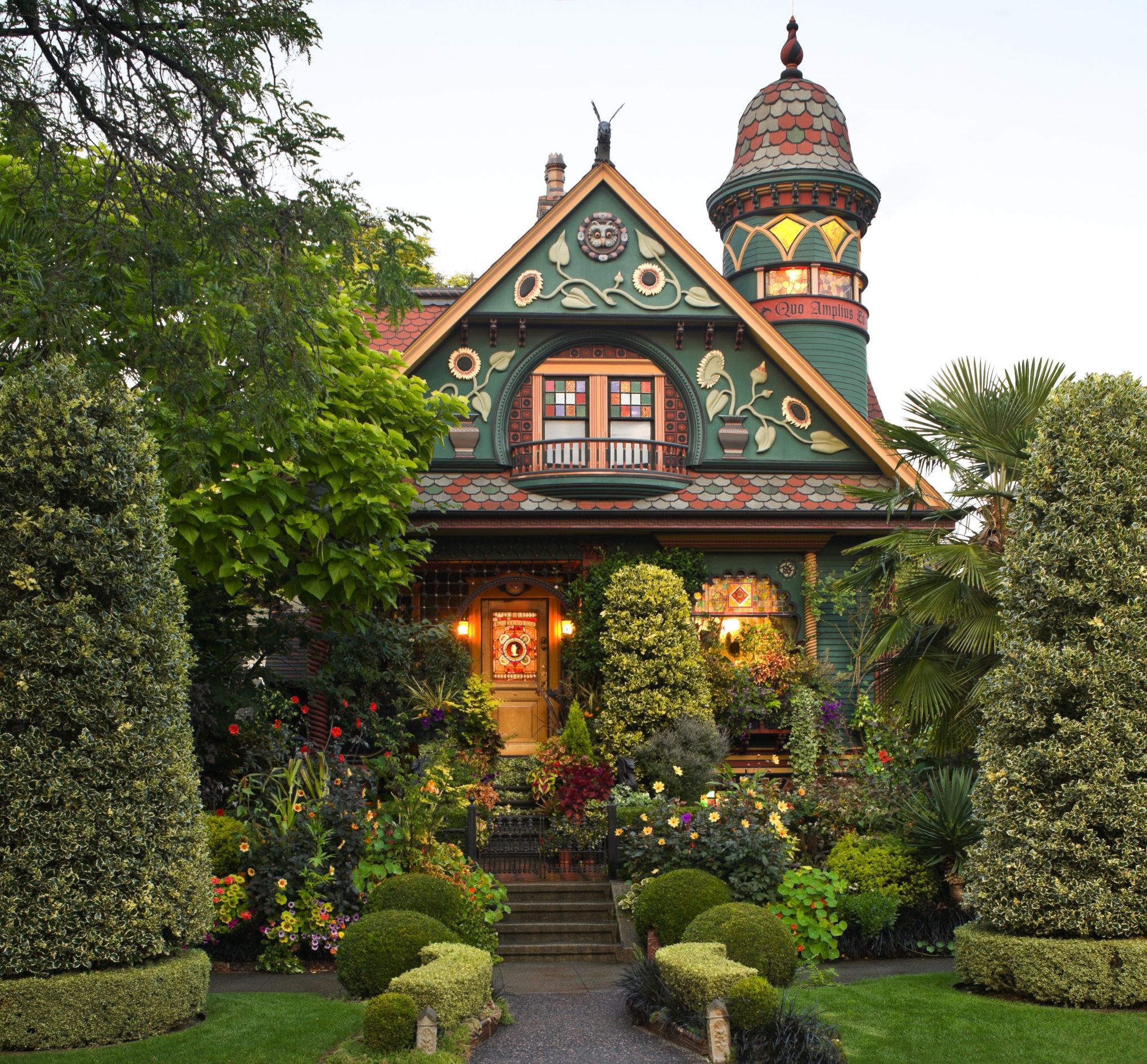This outdoor image showcases an exceptionally well-maintained, Victorian-style house surrounded by a lush, manicured landscape. The home, painted a vivid dark green with red and gold accents, features ornate details including vine and daisy designs adorning the roof and a unique stone lion's face on the upper triangular section. A cylindrical tower with shaded yellow diamond shapes further adds to its character. The front of the house, reminiscent of a fairy-tale dwelling, boasts a circular balcony area and a brown wooden door with an elegant stained-glass window. The approach to the entrance is marked by perfectly round bushes and a dark gray walkway flanked by vibrant flowers. On either side of the house, tall, cylindrical bushes and larger trees with cascading green leaves complete the picturesque scene, making it reminiscent of a setting one might find in Disneyland. The windows, adorned with a mosaic of red, orange, and white cubes, add to the home's colorful and whimsical charm.